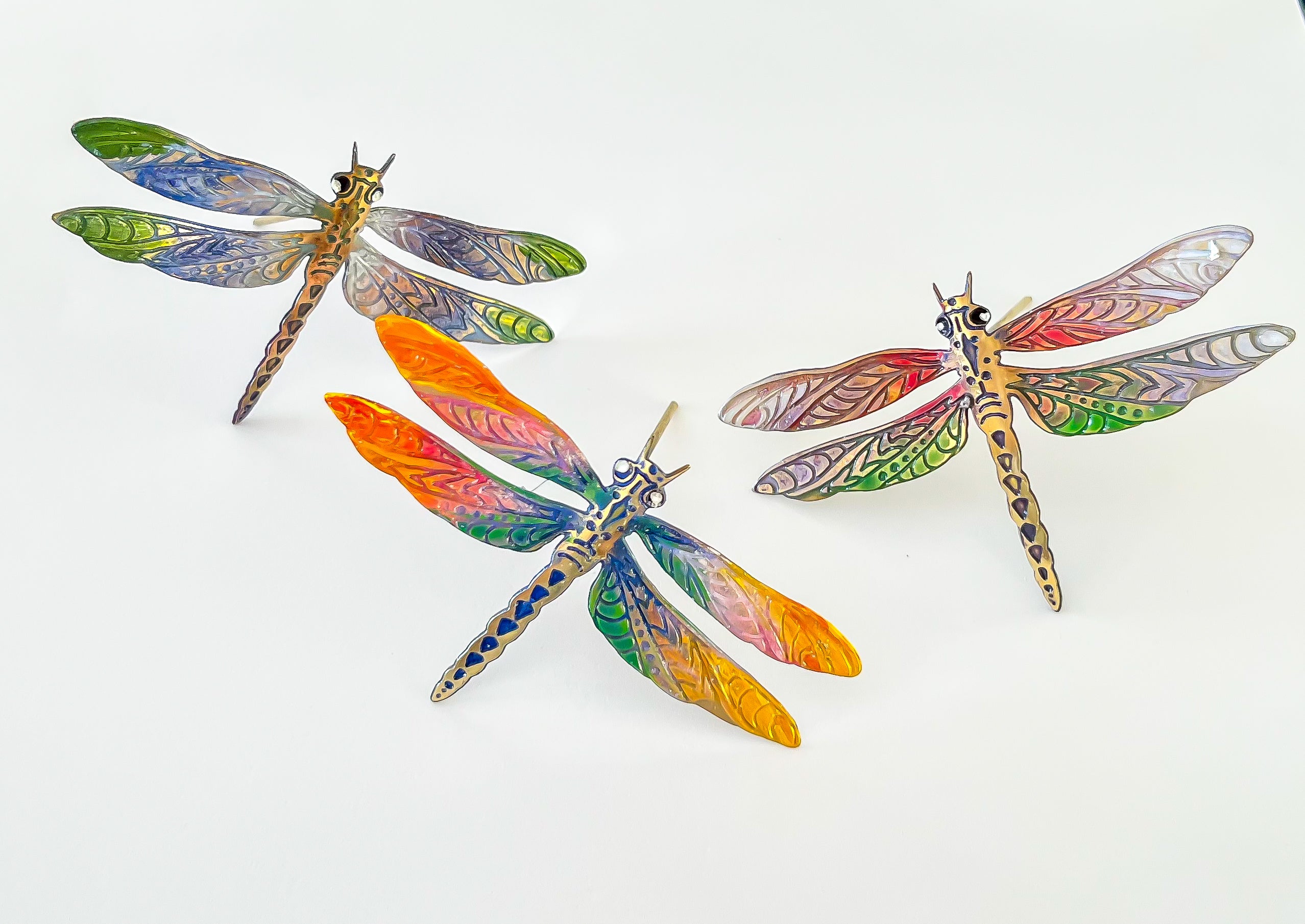The image showcases three vividly colored dragonfly sculptures, each made of plastic or metal, set against a stark white background. The dragonflies, arranged in a triangular formation, exhibit a range of hues across their segmented bodies. The top left dragonfly features wings in shades of green, blue, and a dominant purple, with its body alternating between yellow and hints of green. The central dragonfly boasts an even brighter palette with pink, green, and yellow wings, alongside vivid orange and red hues, contrasted by a body primarily in yellow with accents of blue. The rightmost dragonfly stands out with primarily red and pale yellow wings, accented with green and some orange, and its body shows yellow with traces of pale purple. All three dragonflies share a similar structural design: straight-line middle bodies adorned with triangular markings on the tails, large eyes, and two antennae. These colorful insect sculptures are a vibrant and cohesive set captured on a minimalistic white backdrop.